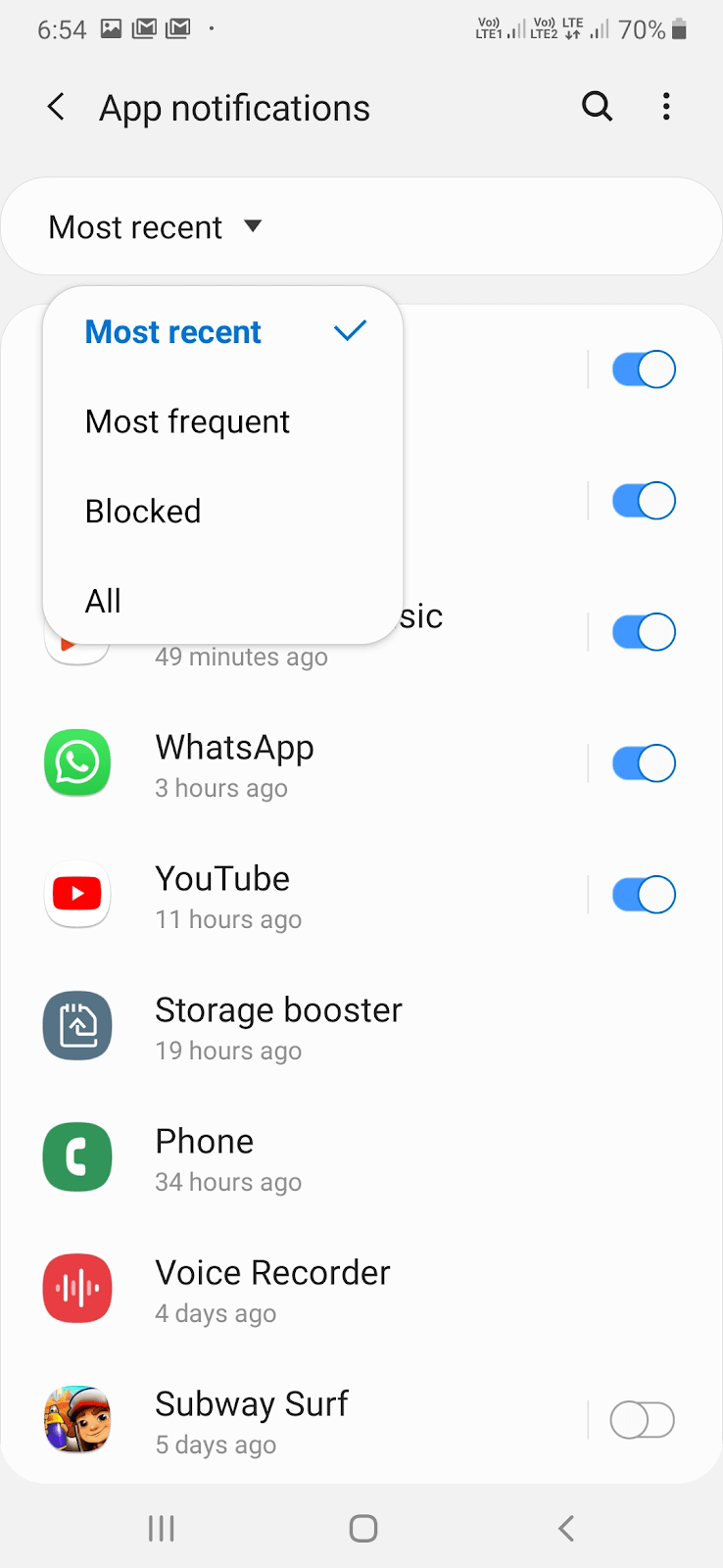The screenshot captures the display of a phone at 6:54 AM, as shown by the time on the top bar. The status bar includes indicators such as a picture icon, several mail icons, Wi-Fi signal strength at two bars, cellular service signal at two bars, and battery life at 70%.

The screenshot reveals the "App Notifications" settings screen, indicated by a left-pointing arrow for navigation, a search magnifying glass icon, and a three-dot drop-down menu for additional options. The visible section of the screen shows sorting options for app notifications, where "Most Recent" is currently selected, but it can also be sorted by "Most Frequent," "Blocked," and "All."

The top portion of the apps list is partially obscured by the drop-down menu, but the right-hand toggle for enabling notifications is visible. The listed applications include WhatsApp, YouTube, Storage Booster, Phone, Voice Recorder, and Subway Surfers. For Subway Surfers, the notifications are turned off, while the prior apps do not display an option to turn notifications on or off within this view.